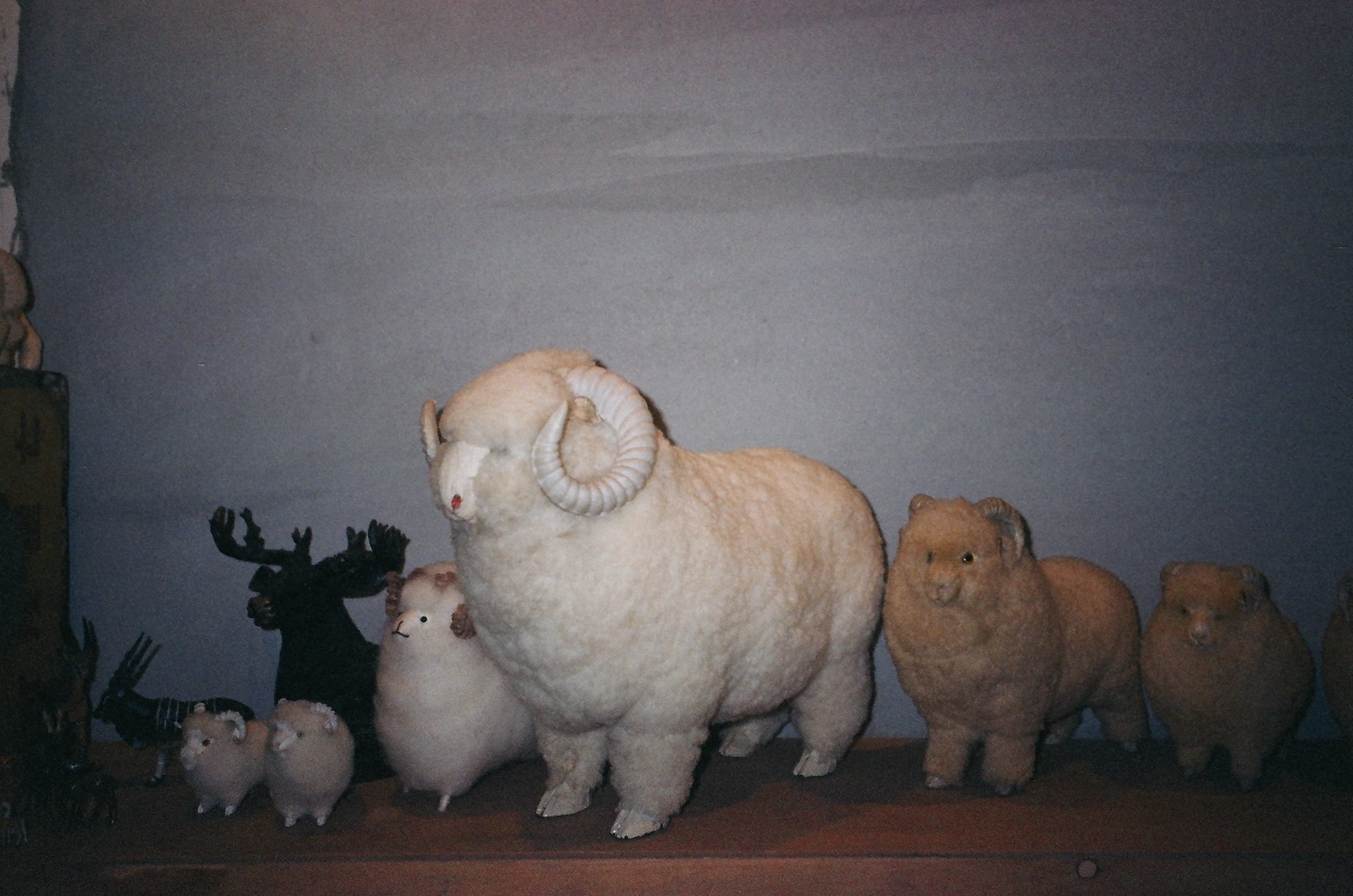This photograph showcases a diverse collection of sheep figurines meticulously arranged on a dark brown wooden shelf against a slate grayish-blue background. The centerpiece of the collection is a large, fluffy white sheep with rounded white horns, facing towards the left. Flanking this central figure are two smaller sheep to the right, both adorned in a beige color with painted eyes, a nose, and a mouth, and the rightmost one being the smallest in size. On the left side of the large sheep, there are three more figurines: a medium-sized white sheep followed by two smaller ones that mimic the largest sheep in their fluffy appearance and rounded horns. The two smallest on the left are woolen longhorn sheep, distinguished by their detailed painted facial features. Additionally, partially obscured within the arrangement is an image of a moose and other wooden animal figures, adding to the eclectic nature of the display. The figurines rest on a reddish-brown cloth that complements the wooden shelf, collectively creating an endearing and well-curated whimsical scene.